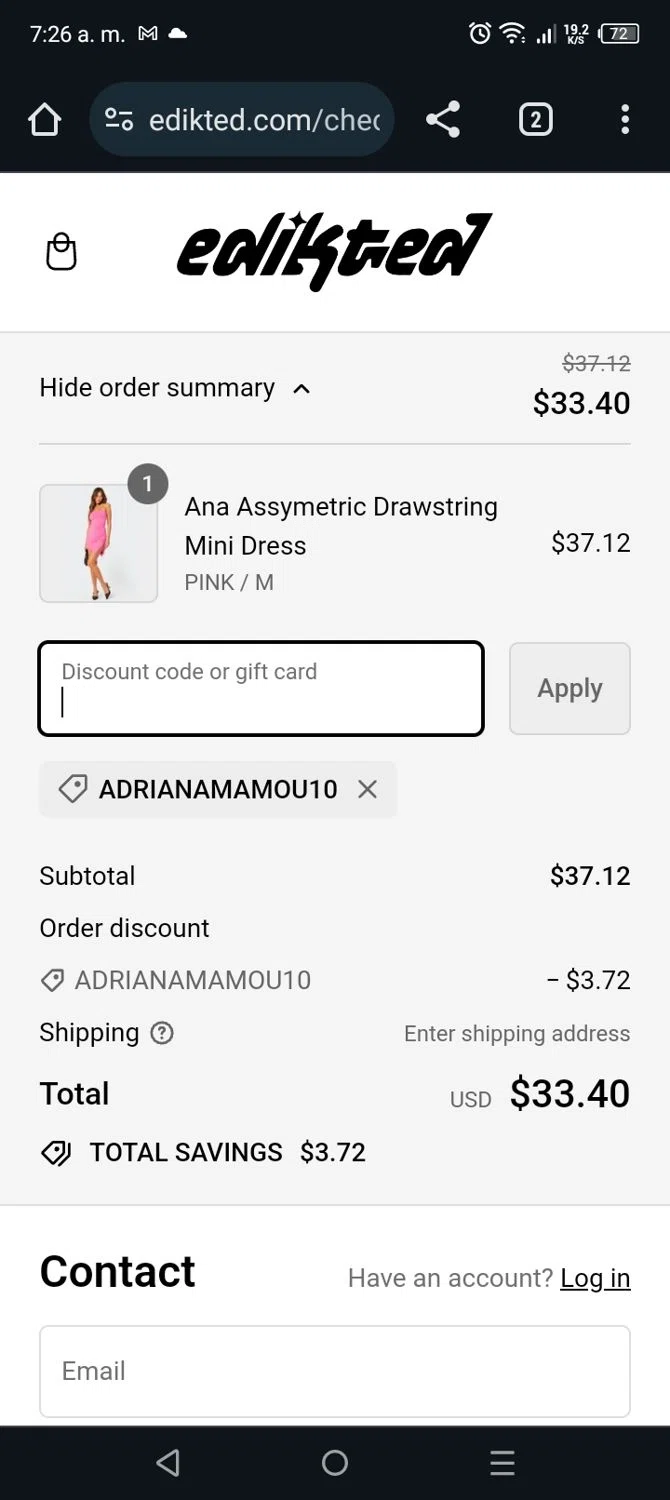The image features a smartphone screen displaying a website. At the top, a black banner shows the time as 7:26 AM, along with icons for an alarm clock, Wi-Fi signal, cellular signal strength, and battery level at 72%. The browser is opened to the website edikted.com, where the user is in the process of making a purchase. The page prominently displays the company name and an order summary. The ordered item is an Anna Asymmetric Drawstring Mini Dress in pink. The original price of the dress was $37.12, but a discount code "AdrianNamu10" was applied, reducing the price by $3.72. The final total is $33.40. At the bottom of the screen, there is a "Contact" button and a prompt for users to log in with their email if they already have an account.